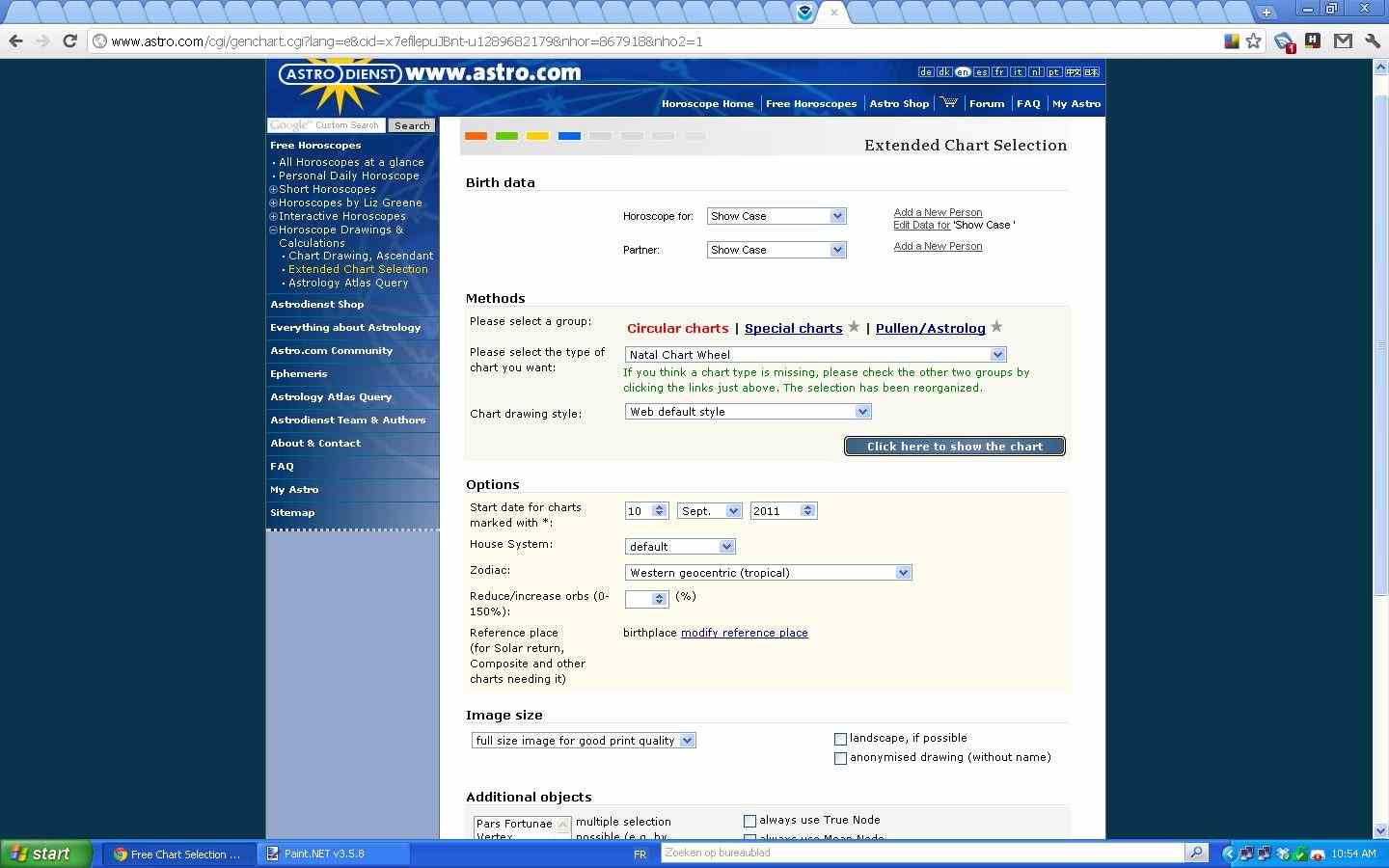In this image, we are viewing a website called www.astro.com. The website is not for a dentist but features a header with the term "Dienst," which translates to "service" in English. In the top left corner, there is a yellow icon resembling a snowflake. The website's interface prominently features very small black text in specific areas.

On the left side of the screen, five main categories are listed: Birth Data, Methods, Options, Image Size, and Additional Objects, each providing various fields for user input. Above these categories is a search bar. The background of the upper section of the site is blue, while the bottom section is gray. The extended chart selection option is located on the top right corner of the interface, with six white categories above it against the blue background.

The outer edges of the website's screen have a very dark blue, almost black background. The top of the page includes a URL bar and a white search bar, separated by thin lines in a light blue section. Additionally, the top right corner features a regular blue color, and at the bottom left of the computer screen, you can see two tabs and the start button, indicating this is a screenshot taken from a Windows operating system.